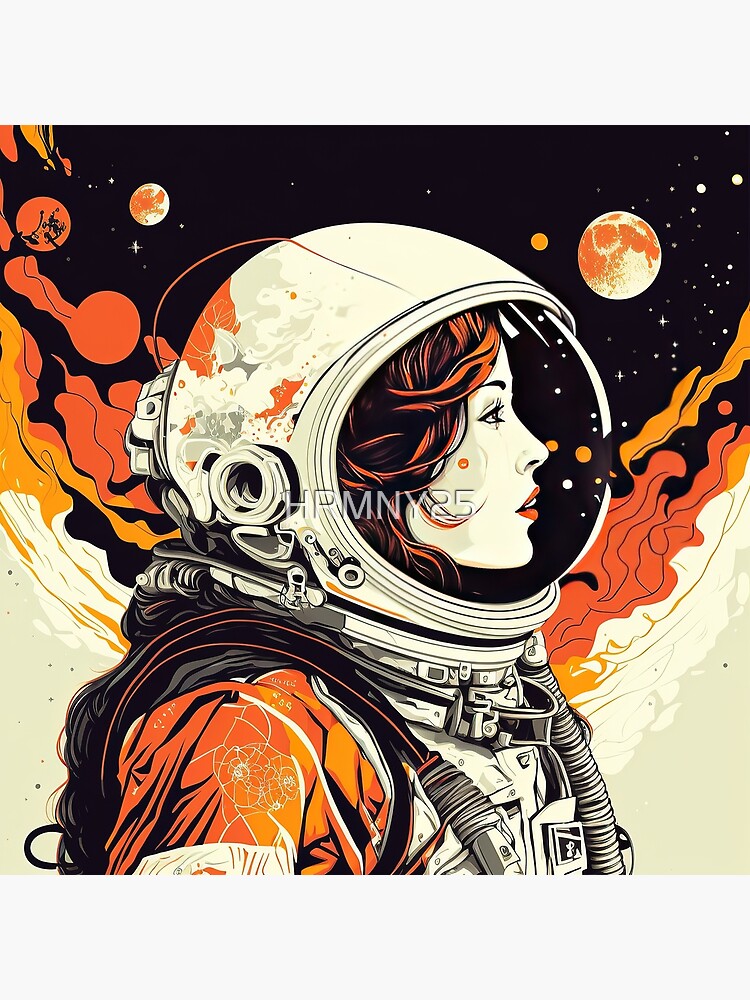This illustration, which has a poster-like style, features a female astronaut depicted in a dynamic side profile. She wears a traditional space helmet with a clear visor, framing her reddish-brown and black hair, and red lipstick. Her space suit is predominantly white, accented with vivid orange sleeves that complement her overall appearance. The background behind her is a vibrant depiction of space, featuring a black sky studded with stars of varying sizes and two detailed planets with visible craters and terrain. Interspersed among the celestial bodies are abstract, lava lamp-like shapes in hues of red, orange, and yellow, mirroring the colors of her suit. The design also includes some text, "H-P-M-N-Y 25," though its significance remains unclear. The scene is highlighted by the burnt orange, mustard yellow, and white tones, creating a cohesive and striking visual narrative.